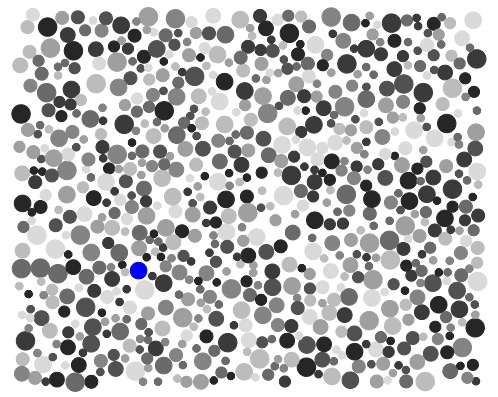The image is a digital artwork consisting of numerous small circles varying in size, predominantly in shades of black, dark gray, light gray, and nearly transparent. These circles are scattered randomly throughout a slightly less-than-square rectangular canvas without any discernible pattern or border. The artwork includes one striking larger dot in the bottom left quadrant, which stands out in a bright blue hue, drawing the viewer's eye amidst the monochromatic array of dots.